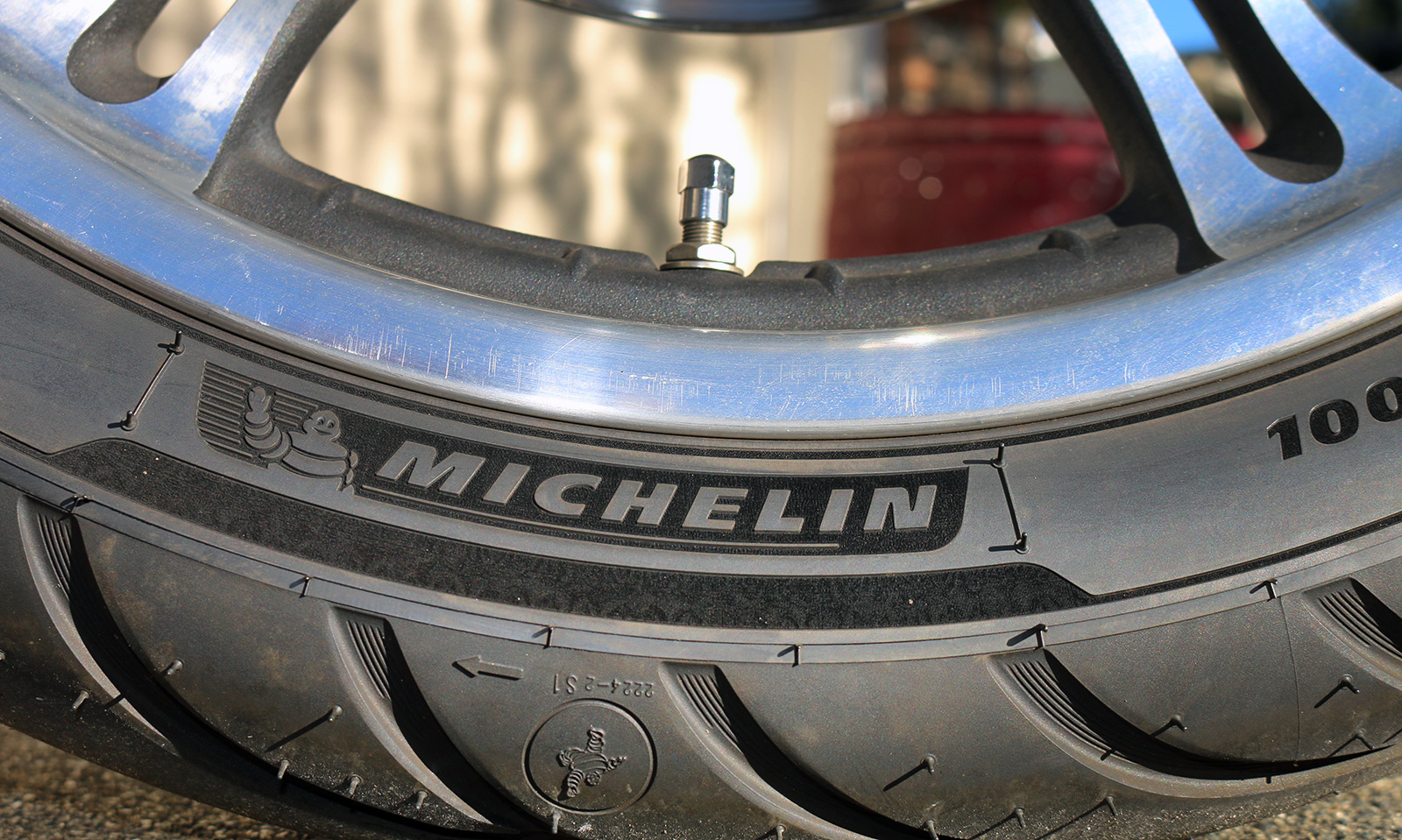This is a close-up photograph of the lower center section of a Michelin tire mounted on a chrome rim. The black tire features significant tread and still has the small rubber nubs indicating it's new. The Michelin logo is prominently displayed on the side, accompanied by the smiling Michelin Man with his right arm raised in a wave. The numbers "2224-281" and "100" are visible on the tire surface. The rim is polished chrome, with normal wear and scratches, and has metal spokes creating open sections through which the blurry, out-of-focus background is visible. The tire valve, capped and hexagonal-topped, is centered in the upper part of the image, and a dark red object in the distant background hints at a possible showroom setting.